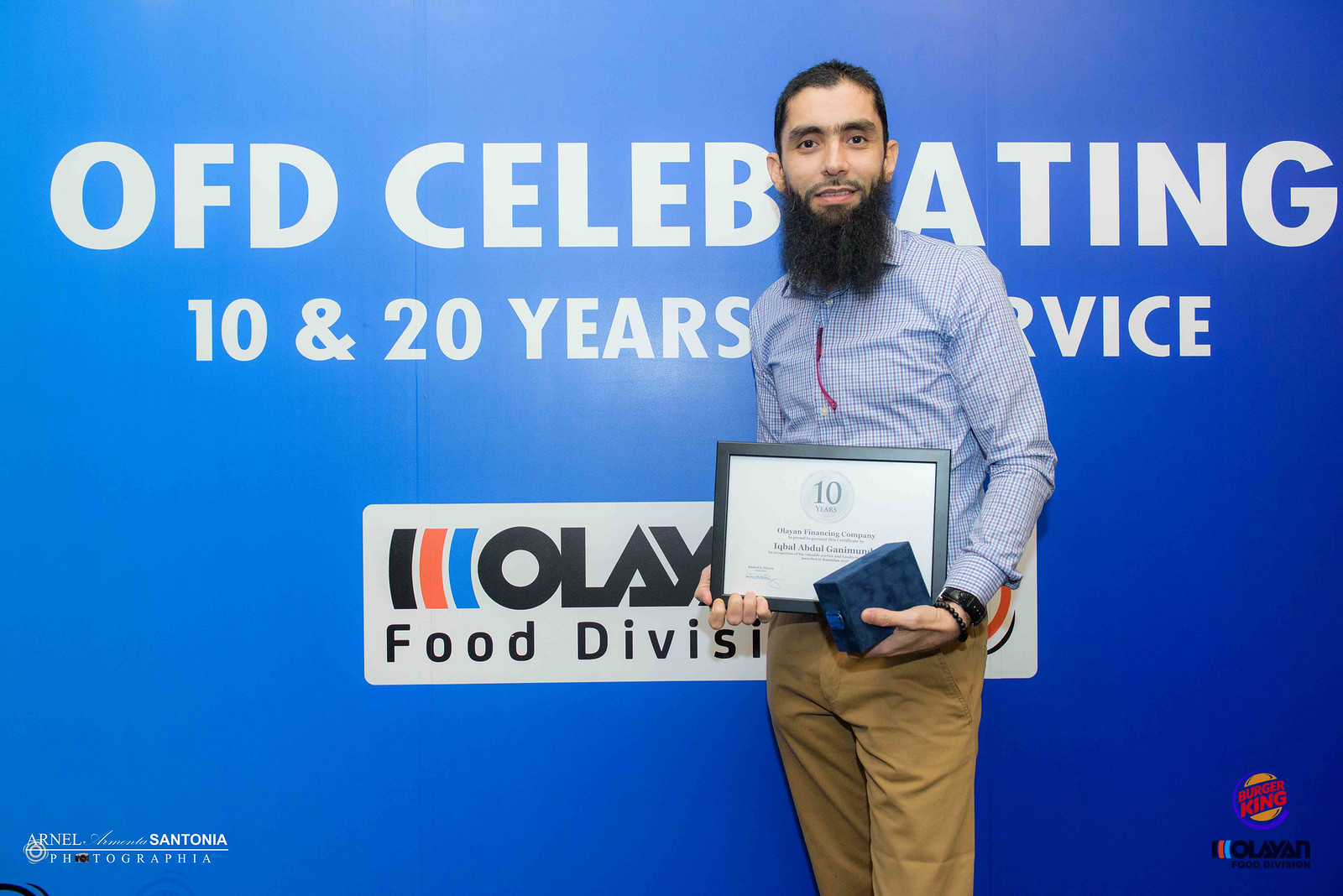In this image, a man is posing in front of a blue backdrop with large, white capital letters that read "OFD Celebrating 10 and 20 Years of Service." The backdrop fades from dark blue to light blue. Below the text is a white rectangle containing a logo and text in red, blue, and black, partially obscured by the man, but you can make out "food division" and "OLA." The man, situated in the right two-thirds of the image, is wearing a blue and white checked button-down shirt with khaki pants. He has a long black beard and is smiling, holding a black-framed certificate in one hand, which appears to indicate "10 years," and a blue box in the other hand, likely a gift. He is also wearing a watch and bracelets. In the bottom right corner of the image, there's a Burger King icon, and the bottom left corner has text that includes "Arnell Photography" and "Santona."